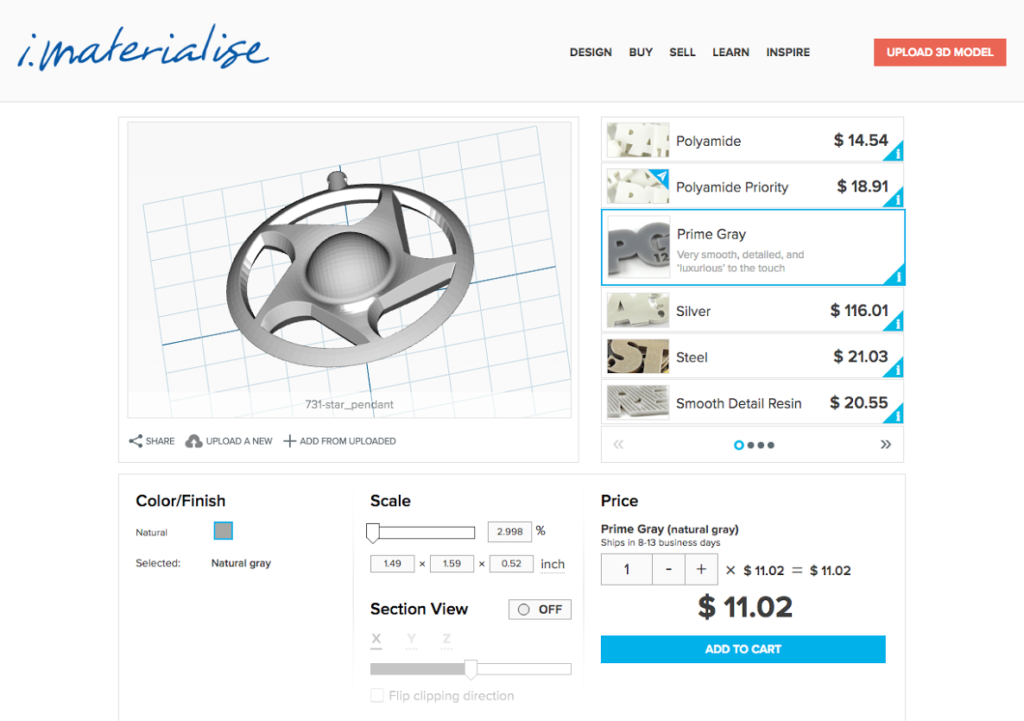The image showcases the Materialize website, featuring its branding and interface elements prominently. At the top, a black banner displays the stylized logo "i.m-a-t-e-r-i-a-l-i.," where the final letter could be interpreted as either a 'Z' or an 'S.' To the middle right of the banner, there are navigational options labeled "Design, Buy, Sell, Learn, Inspire." Further right, an orange rectangle labeled "Upload 3D Model" stands out.

Beneath the banner, the central visual element resembles a hubcap— a circular design with star-like shapes having curved ends that radiate from the center. Directly below this image, a grid layout is visible, followed by icons for sharing, uploading, and adding files.

The section below features interface controls for customizing options. The "Color / Finish" section shows "Neutral," with "Selected: Neutral Gray" specified alongside a gray box icon. The "Scale" option is shown minimized. Further down, the "Section View" option indicates it's turned off. The "XYZ" bar is positioned in the middle, while for pricing, it displays "1 Folded 1102." Lastly, a prominent "Add to Cart" button is located at the bottom.